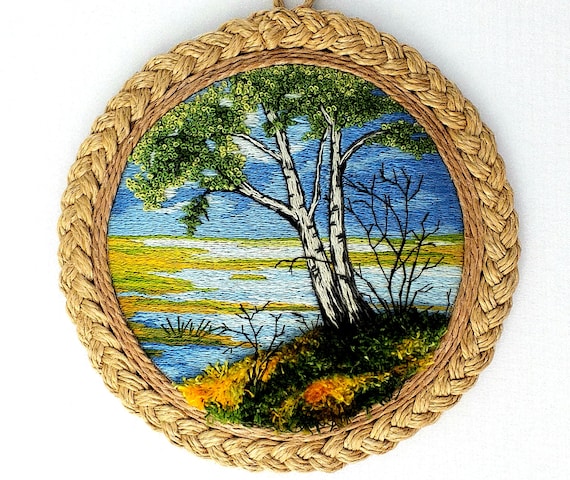This photograph depicts a stunning piece of detailed embroidery with a circular woven rope frame in light brown, adding to its rustic charm. The artwork showcases a beautifully textured scene of a birch or aspen tree with striking white bark and lush green leaves. The tree leans slightly to the left, rooted in a small, shaded hill adorned with green grass and subtle hints of yellow. In the serene background, a light blue sky with scattered white clouds fades into a watery area, possibly a lake or river with greenish land inlets. The intricate stitches create a rich, textured effect, making the leaves appear curly and the grass almost shaggy. This handmade piece, photographed against a plain white background, combines various embroidery techniques, capturing nature's serenity and attention to detail in a manner reminiscent of a painting.